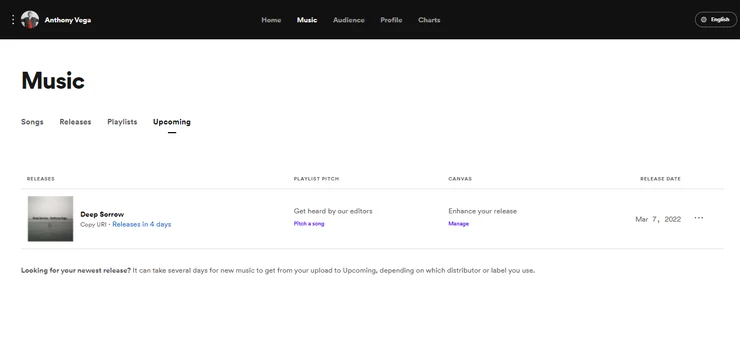Screenshot Description:

The screenshot appears to be from a music sales or streaming site. At the top, there's a black bar containing the user's profile in the upper left-hand corner, showing the logged-in user as Anthony Vega. 

Below this is the main menu bar with several items: Home, Music, Audience, Profile, and Charts. The language selected for the site is English. In this instance, the 'Music' section is selected, as indicated by its highlighted state.

The main content area of the screen focuses on the 'Music' section, marked by a large title that says "Music." Below this title, a smaller menu is present featuring options such as Songs, Releases, Playlists, and Upcoming. The 'Upcoming' tab is currently selected.

Directly under the 'Upcoming' tab, there is a listing for an upcoming release, presumably belonging to the artist associated with the account. The details provided include:

- Release Title: "Deep Sorrow"
- Album Cover Art: Displayed next to the title
- Release Countdown: "Releases in four days"
- Additional Feature Options: 
  - Playlist Pitch: Get heard by our editors
  - Canvas: Enhance your release
- Stated Release Date: March 7, 2022

Overall, it seems like this is a platform designed for music artists to manage and promote their album releases.